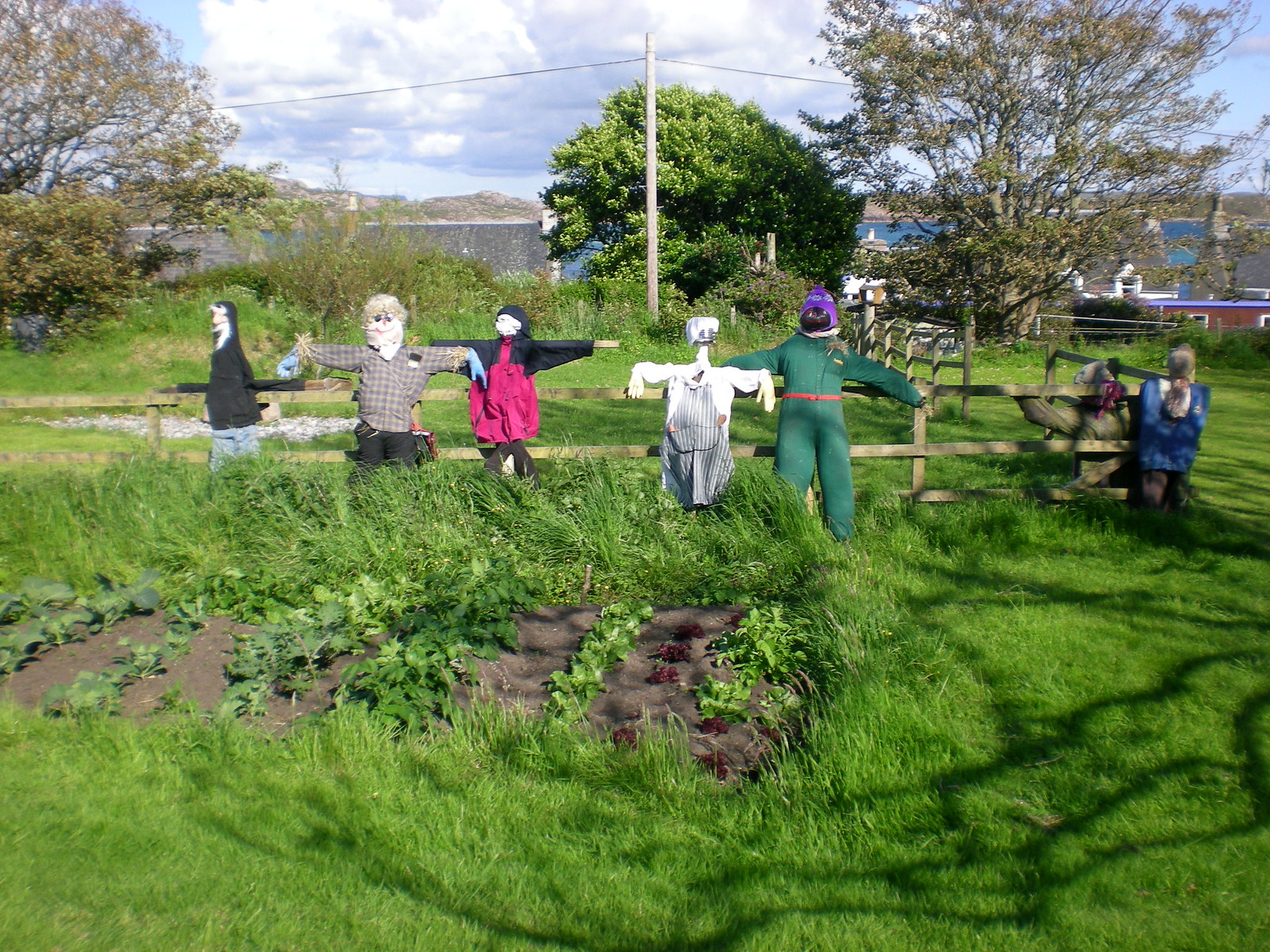This photograph captures a rustic outdoor scene featuring a small garden plot encircled by a grassy lawn, some of it overgrown and wild. The garden itself shows rows of produce with a variety of leaves in shades of green and reddish-purple. Flanking the far side of the garden is a wooden fence, and standing prominently against it is a line of six scarecrows, each uniquely dressed and positioned with outstretched arms. Their outfits range in style and color, including a green jumpsuit, a striped apron, a black shirt with dark red overalls, a checked shirt with blue gloves, a red and black windbreaker, and blue striped coveralls paired with a white shirt. Additionally, another scarecrow is seen blending into the background with tan-colored attire. Each scarecrow contributes to the scene's eclectic and whimsical charm. In the distance, a backdrop of trees and power lines frames the garden, stretching out towards a calm body of water, beyond which lie hills under a sky dotted with clouds. The serene landscape is further complemented by the presence of houses along the water's edge.